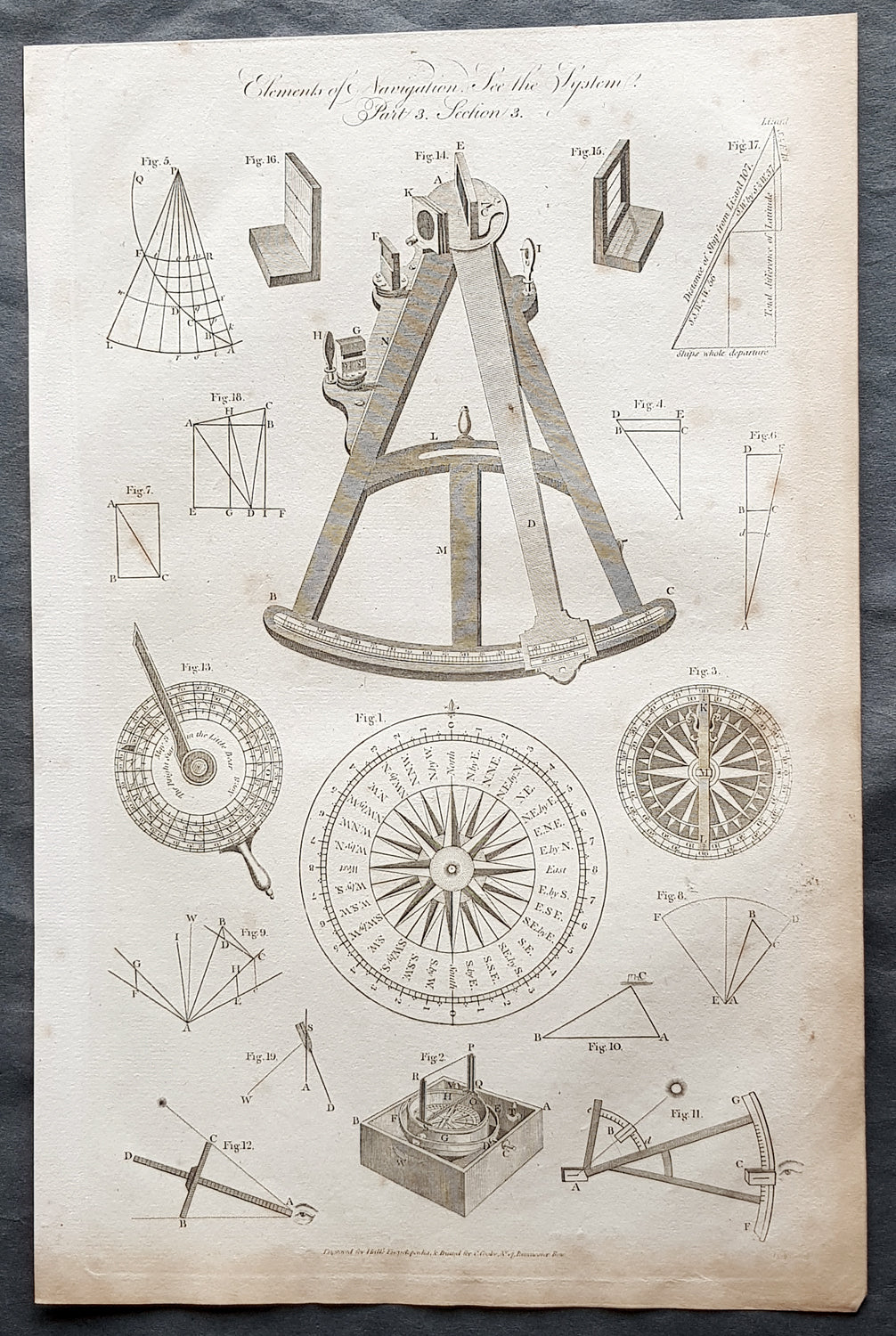This black and white historical engraving from 1791 features a series of detailed diagrams, illustrations, and drawings of measuring instruments and navigational tools. The centerpiece is a large compass labeled “Figure One,” flanked by two smaller compasses: “Figure Three” on the right and “Figure Thirteen” on the left. Above these compasses is a prominent drawing of a sextant with a triangular shape, surrounded by smaller diagrams and lines that illustrate its function. Calligraphy-type writing at the top reads "Elements of Navigation, See the System." The page includes fifteen figures depicting various measurement devices, which were used for gauging wind, temperature, sound, and size. Additional illustrations beneath the compasses and sextant show different shapes, angles, and sections, including triangular drawings adorned with numbers and letters, providing a comprehensive explanation of the mechanics and usage of these historical tools.